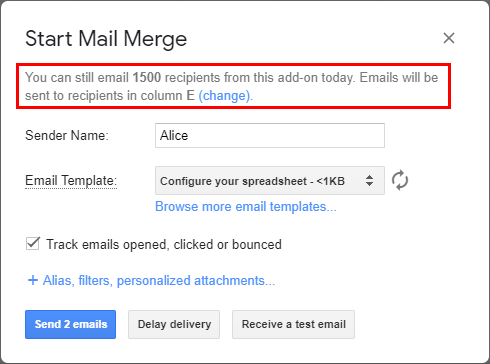This image showcases a "Start Mail Merge" interface prominently displayed at the top left corner in bold black font, with each word capitalized. The text is highlighted by a red box, emphasizing the function. Below the highlighted text, a gray font message explains, "You can still email 1,500 recipients from this add-on today. Emails will be sent to recipients in column E." There is an option in parentheses labeled "change," placed beneath the main message.

The interface further reveals the sender's name as "Alice." Below this, there is a section for the email template, labeled "Configure your spreadsheet," and an additional note indicating that the template size is larger than one kilobyte. Another option, "Browse more email templates," is available beneath that.

Further down, several checkboxes are visible, one of which is checked, indicating the option to "Track emails opened, clicked, or bounced." Lastly, there is a prominent "Send Emails" button, ready for initiating the mail merge process.